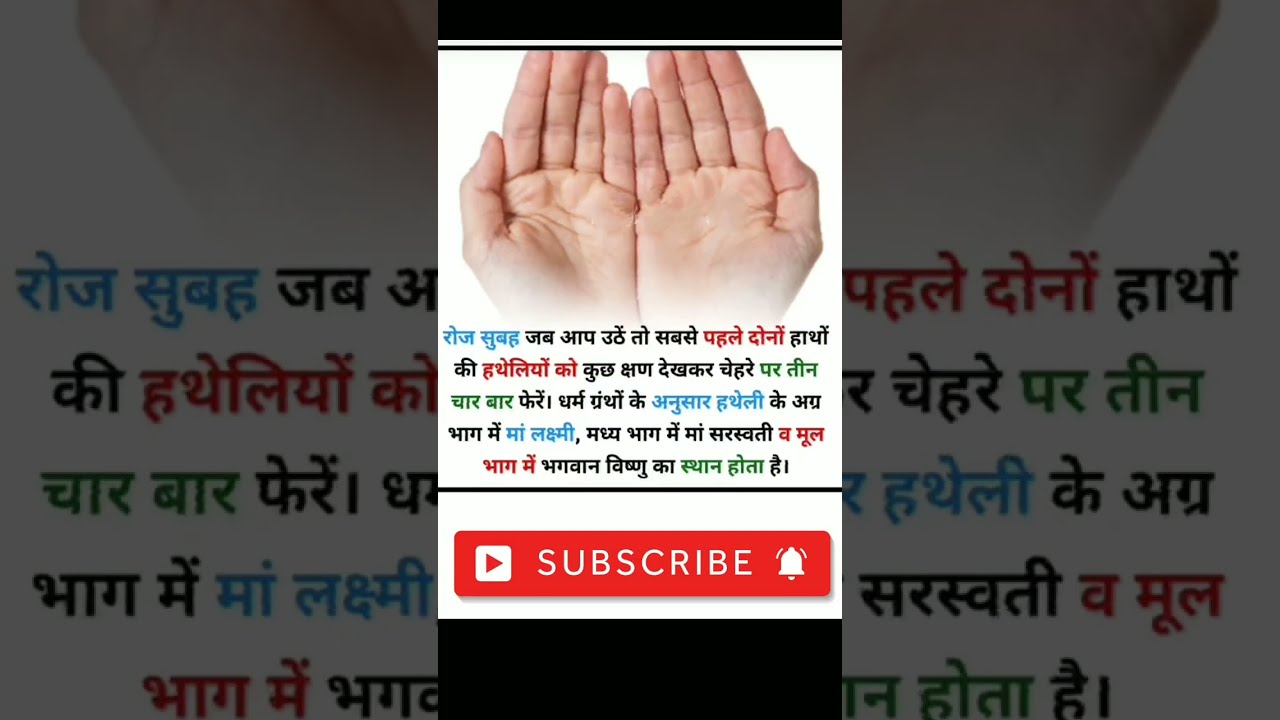The image features two hands, likely Caucasian, with palms facing up and pinky fingers touching, centered on a white background. The layout includes three vertically aligned rectangles: the central one displaying the full image, while the left and right rectangles present zoomed-in portions of the hands, with slightly darker lighting. Intricate text in a foreign language, primarily black but interspersed with blue, red, and green characters, overlays the image. Below the text, a prominent red rectangle contains a white "subscribe" text flanked by a YouTube play button on the left and a notification bell on the right.